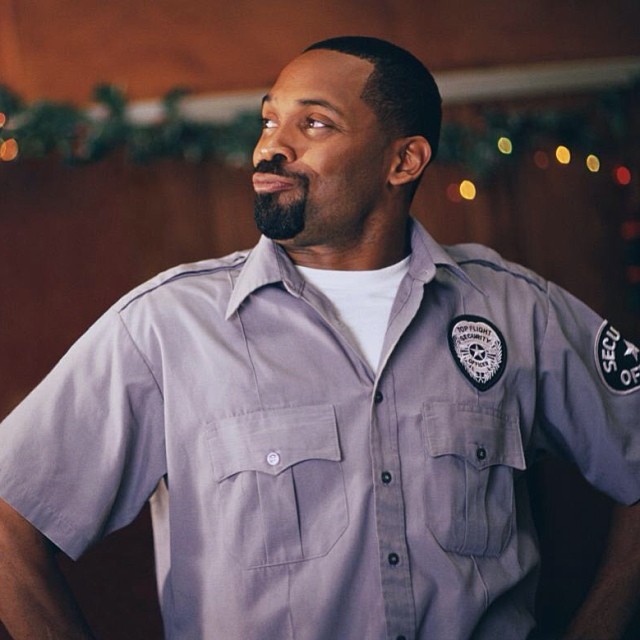The image features a confident African-American man, dressed in a Top Fly Security uniform. He is clad in a slightly wrinkled, short-sleeved, button-down collared shirt of a light greyish-blue hue, over a white undershirt. The shirt bears a distinct badge patch on the right chest and a security patch on the right arm sleeve. He has dark brown skin, a short buzz cut, and well-trimmed black facial hair, including a slight mustache and goatee. The man stands with his hands on his hips, looking smugly to his left, with a slight pout. The background is blurry, showcasing a brown wall adorned with green Christmas tinsel and lights.